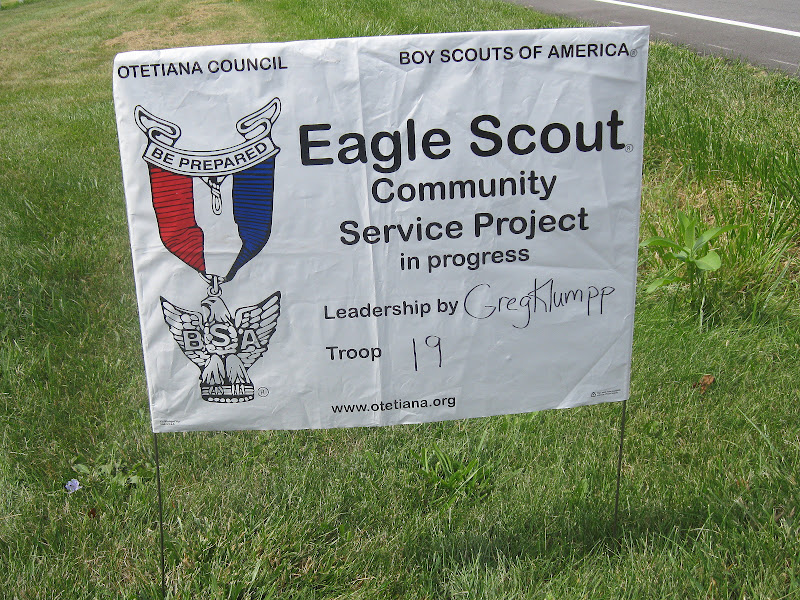The image features a yard sign situated in a grassy area beside an asphalt paved roadway. The sign is supported by two black metal poles embedded in the ground. The rectangular sign has a white background and is made of a material that resembles plastic rather than wood. In the upper left corner, the sign bears the text "O-T-E-T-I-A-N-A Council" in all capitalized black print. Below this, there is a crest with a banner that reads "Be Prepared" in black text. The crest also features a red, white, and blue shield, divided by vertical lines, with a forward-facing eagle positioned below. The eagle, shown in profile with outspread wings, has the initials "B-S-A" in front and stands on a black pedestal.

To the right of the crest, in the upper right corner of the sign, "Boy Scouts of America" is written in black, capitalized letters. Below this, in larger black print, are the words "Eagle Scout." Further down, "Community Service Project" is printed, followed by "In Progress." Just below, "Leadership By" is printed in black, with the handwritten name "Greg Klump," and "Troop 1919" also handwritten beneath. At the bottom of the sign, there is a printed website URL: www.otetiana.org. The sign is placed in a grassy area punctuated with a few weeds, characterizing its temporary installation nature.